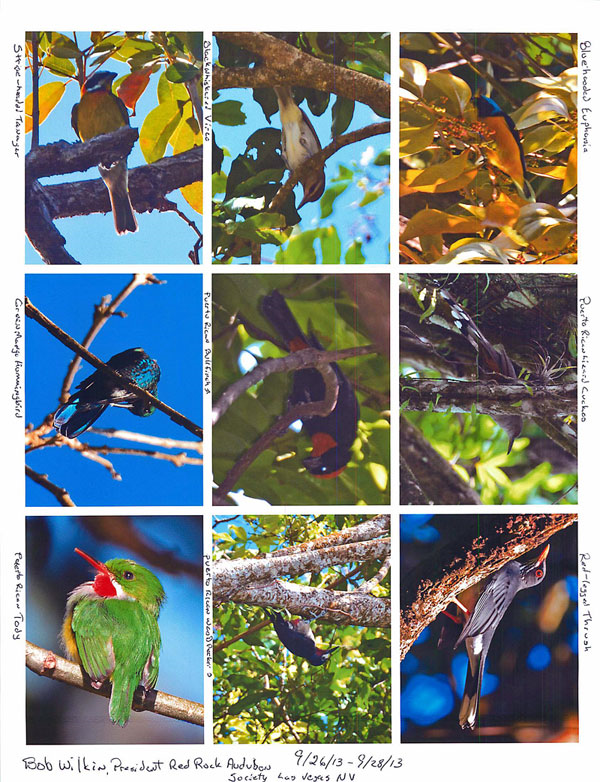This vibrant outdoor montage showcases a collage of nine bird photographs, each meticulously placed in a three-by-three grid. The images, captured under sunlight, feature various birds perched on branches in their natural habitat, providing an intimate and detailed look at their serene resting moments. The birds' colors pop against the vivid backdrop of greens and blues, enhanced by the occasional red, purple, brown, and yellow hues. Each bird is uniquely colored, ranging from a striking yellow and black bird to a white and brown bird, and even a small green bird with a bold red beak. The birds are individually labeled with small text that is hard to read, possibly denoting species and descriptions. The bottom of the montage credits Bob Wilkin, President of the Red Rock Audubon Society, from Las Vegas, Nevada, highlighting his term from September 2013 to September 28, 2013. Every photograph captures the essence of these birds in stillness, providing a captivating glimpse into their outdoor existence.